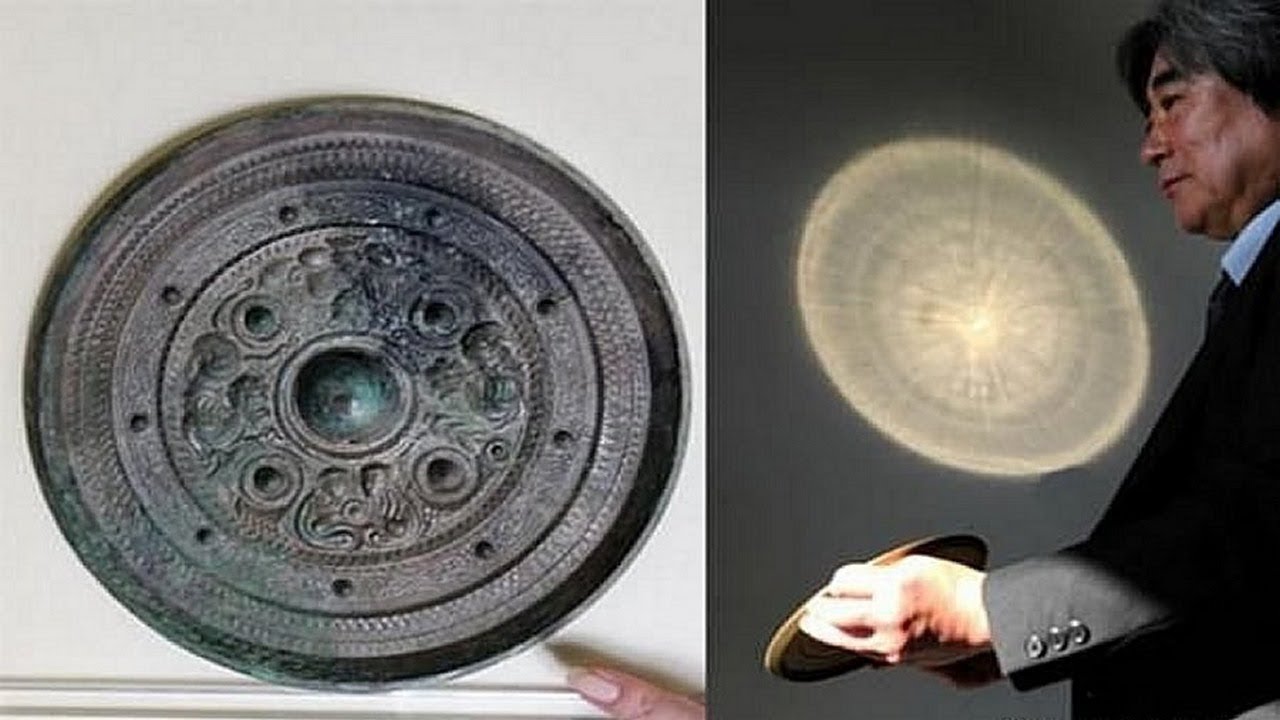The image is divided into two adjacent sections. On the left, there is a large round metallic disc that features intricate detailing, with multiple concentric circular patterns. The disc appears to have a bronze or grayish hue with a turquoise-tinted central hole surrounded by four smaller indentations near the middle. At the bottom right of this section, a woman's finger with a long fingernail points to the disc. On the right side of the image, an older Asian man dressed in a black suit with a white collared shirt is holding the disc. Seen from a side view, he wears a serious expression and appears to be focusing intently on the task at hand. The disc projects a bright reflection onto a surface with a gray background, resembling a spotlight effect.